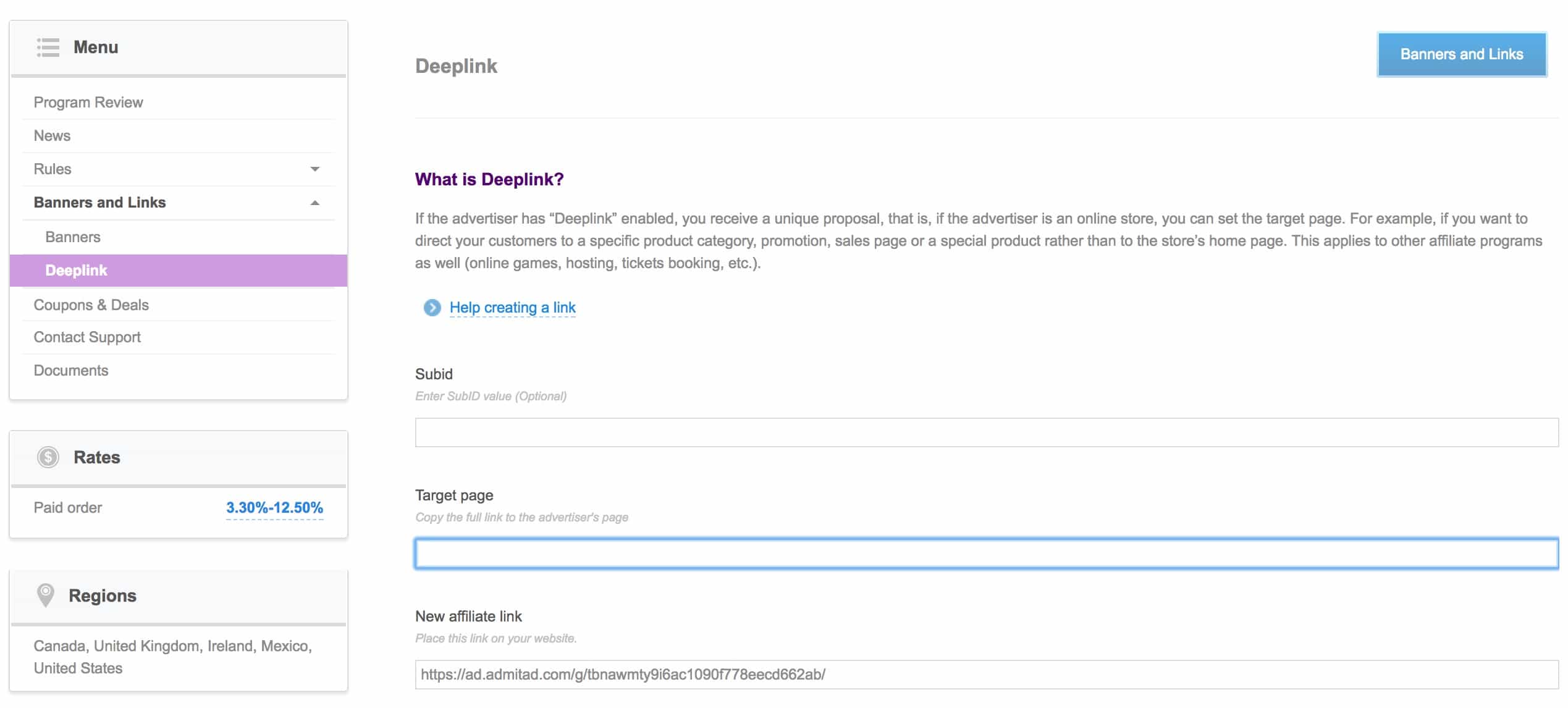This image depicts a detailed interface of an application or website dedicated to deep linking functionalities. On the left side, a vertical menu column lists several options, including "Program Review," "News," "Rules," and "Banners and Links" highlighted in purple. Moving rightward, the central section prominently features a heading labeled "Deep Link." To the far right, there is a prominent blue box containing the text "Banners and Links" in white.

Deep linking enables advertisers to provide unique proposals. For instance, if the advertiser is an online store, deep linking allows directing customers to specific product categories, promotional pages, sales events, or particular products rather than the store's homepage. This functionality is applicable across various affiliate programs, including online games, web hosting services, and ticket bookings.

The image also includes guidance on creating a link, with information and instructions extending downward towards the bottom of the interface.